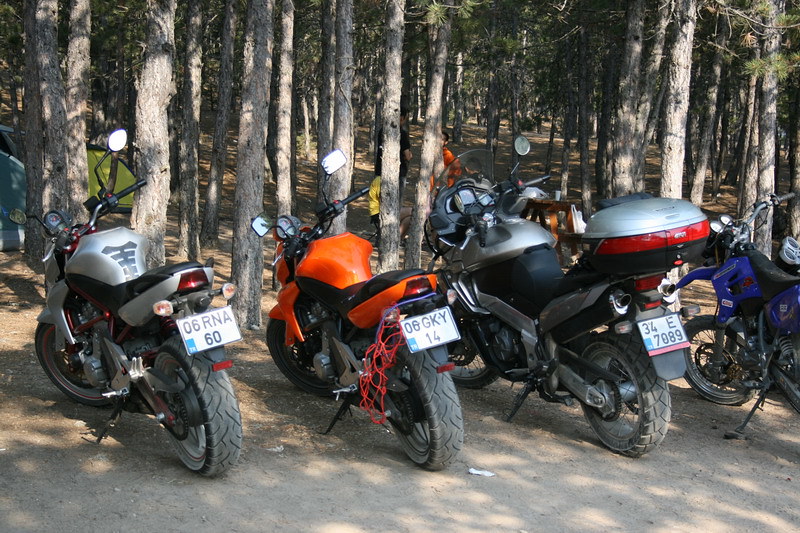This photograph captures a detailed scene of four motorcycles parked diagonally and very close together, about a couple of feet apart, on a dirt road or dirt lot in front of a tree line in what appears to be a park or wooded area. The motorcycles are positioned with their fronts facing the woods, where you can see tall, grayish trunks of trees suggesting they might be fir trees. The leaves are high up and mostly out of the frame. 

Starting from the left, the first motorcycle is silver and black, described as very short with a single rider's seat, high side view mirrors, and small wheels. Its license plate reads "06RNA60." The second motorcycle is orange, sitting low to the ground, with a longer body compared to the first. It has orange plastic netting hanging off the back, high rectangular side view mirrors, and the license plate "06GKY14." 

The third motorcycle is significantly larger, gray with black seats, and equipped with a large case on the back that seems suitable for storage, possibly for camping gear given the environment. It also features a windshield and what appears to be a navigation system. Its license plate is "J4E7089." In front of this motorcycle, a picnic table with a cup on it is noticeable, along with people, possibly a father and two sons, standing behind the trees. 

The final motorcycle is blue and smaller, similar in style to the first two, but less visible in the image. Small wheels and a single seat hint at its compact nature. The setting includes additional elements, such as a blue and a green tent in the background, suggesting that the motorcyclists may be camping in the area.